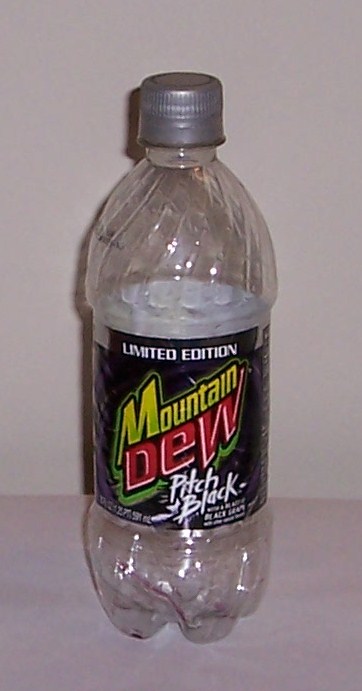A detailed photograph captures an empty, 12-ounce screw-top bottle of Mountain Dew's limited edition "Pitch Black" flavor. The distinctive, eye-catching label features a predominantly black wraparound design. The iconic Mountain Dew logo appears prominently in a playful, cartoon-style font, with the words "Mountain" and "Dew" rendered in rounded, red letters accented with white highlights. Above the logo, the "Limited Edition" label is clearly visible, while the words "Pitch Black" are displayed in an eerie, slasher-inspired white font against a black background, adding a dramatic and intense visual effect.

The bottle itself is shorter and more robust compared to the typical 16-ounce variety, emphasizing its unique size. Its silver screw-top cap has been securely replaced on the empty bottle, which stands upright on a gray shelf. The background of the image is an off-white hue, allowing the bold colors and striking design of the bottle to stand out prominently.